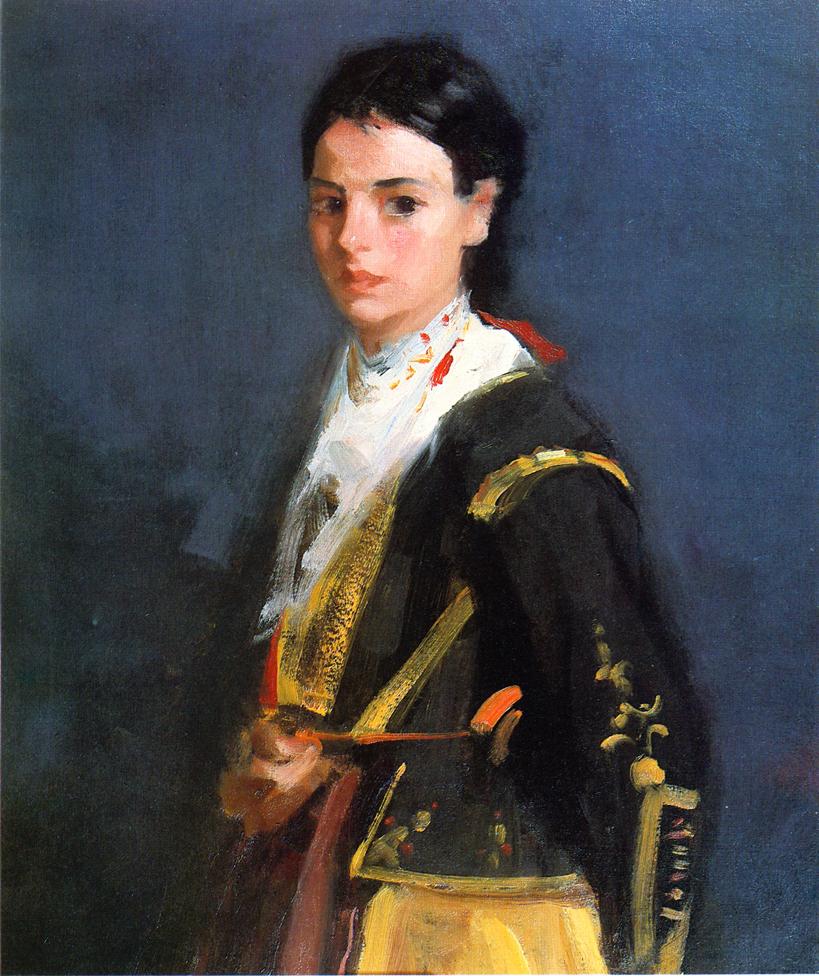This is a detailed painting of a youthful individual with an androgynous appearance, though possessing traits that lean toward feminine. The figure has striking black hair, dark eyebrows, and large, expressive black eyes, set against a fair complexion. The person is attired in a distinguished, almost regal ensemble that suggests a military or official standing. They wear a black jacket adorned with elaborate gold emblems and trim, along with a white shirt featuring ornate, fluffy detailing at the neck. The lower garment appears to be gold pants, completing the uniform’s stately look. This attire evokes the grandeur of historical military dress, reminiscent of styles worn by figures like Napoleon. The figure stands in profile, turned to the left, but gazes directly at the viewer with a composed expression. The background is painted in varying shades of blue, adding depth and contrast to the overall composition. The individual might be depicted holding a sword with the right hand, tucked under the left arm, though this detail is somewhat ambiguous. The painting captures an air of youth and distinction, blending elements of historical portraiture with a timeless elegance.